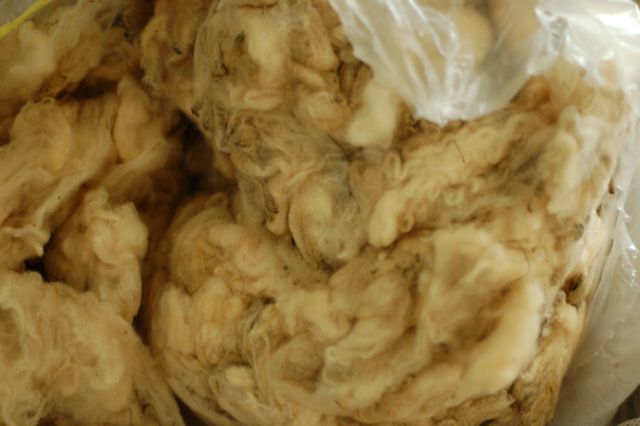This image depicts an extreme close-up of what appears to be very old, matted cotton or unprocessed wool that has been clumped together. The fibers exhibit a dingy yellow to dark brown hue, with a ropey texture creating a swirly pattern throughout the compacted material, which looks dirty and squeezed together. The photograph is slightly out of focus, but the composition clearly shows a torn, mostly opaque plastic bag in the upper right corner, revealing snippets of the fibrous material beneath. In the lower right, the material transitions into a white linen featuring a wobbly diamond stitched pattern, typical of mattress coverings. The overall visual impression suggests the stuffing from an old mattress or an uncarded sheep fleece that has been rolled and shoved into a bag, emphasizing its rugged and unprocessed state.